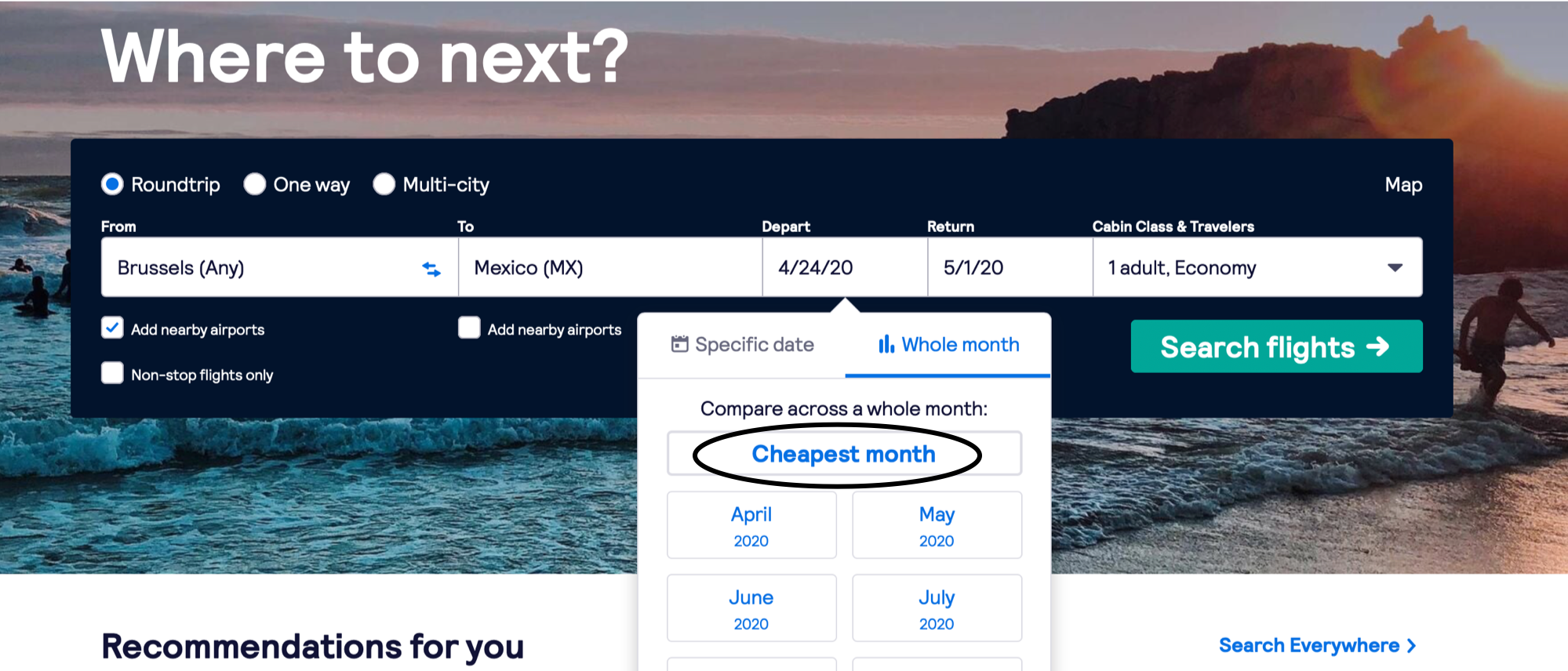The image showcases a vacation travel website interface with a serene beach scene as the backdrop. Dominating the scene is a stunning expanse of vibrant blue water, gently lapping against a sandy shore. On the right side of the image, a man emerges from the water and walks toward the beach, adding a touch of life to the tranquil setting. The horizon in the distance presents a mesmerizing blend where the sky meets the beach, with hues of pink creating a picturesque transition. A mysterious, dark landmass can be seen faintly in the background, adding depth to the scenery.

In bold white lettering, the phrase "Where to next?" takes center stage. Below it, users are given several travel options: Roundtrip, One Way, Multi-City, with Roundtrip currently selected. On the right-hand side, there's an option to view a map. Input fields are labeled From, To, Depart, Return, Cabin Class, and Travelers. The example information is from Brussels to Mexico, with departure on April 24, 2020, and return on May 1, 2020, for one adult. The site has options for including nearby airports, selecting nonstop flights only, and choosing specific dates or a whole month. April, May, June, and July of 2020 are provided as options in a dropdown menu with a white background and blue text.

To the right of the search fields, a prominent turquoise button labeled "Search Flights" in white text and accompanied by a white arrow invites users to start their search. At the bottom of the search window, there are additional options in black and blue text: "Recommendations for you" and "Search Everywhere." The entire interface is designed to be user-friendly, making it easy for travelers to plan their next adventure.